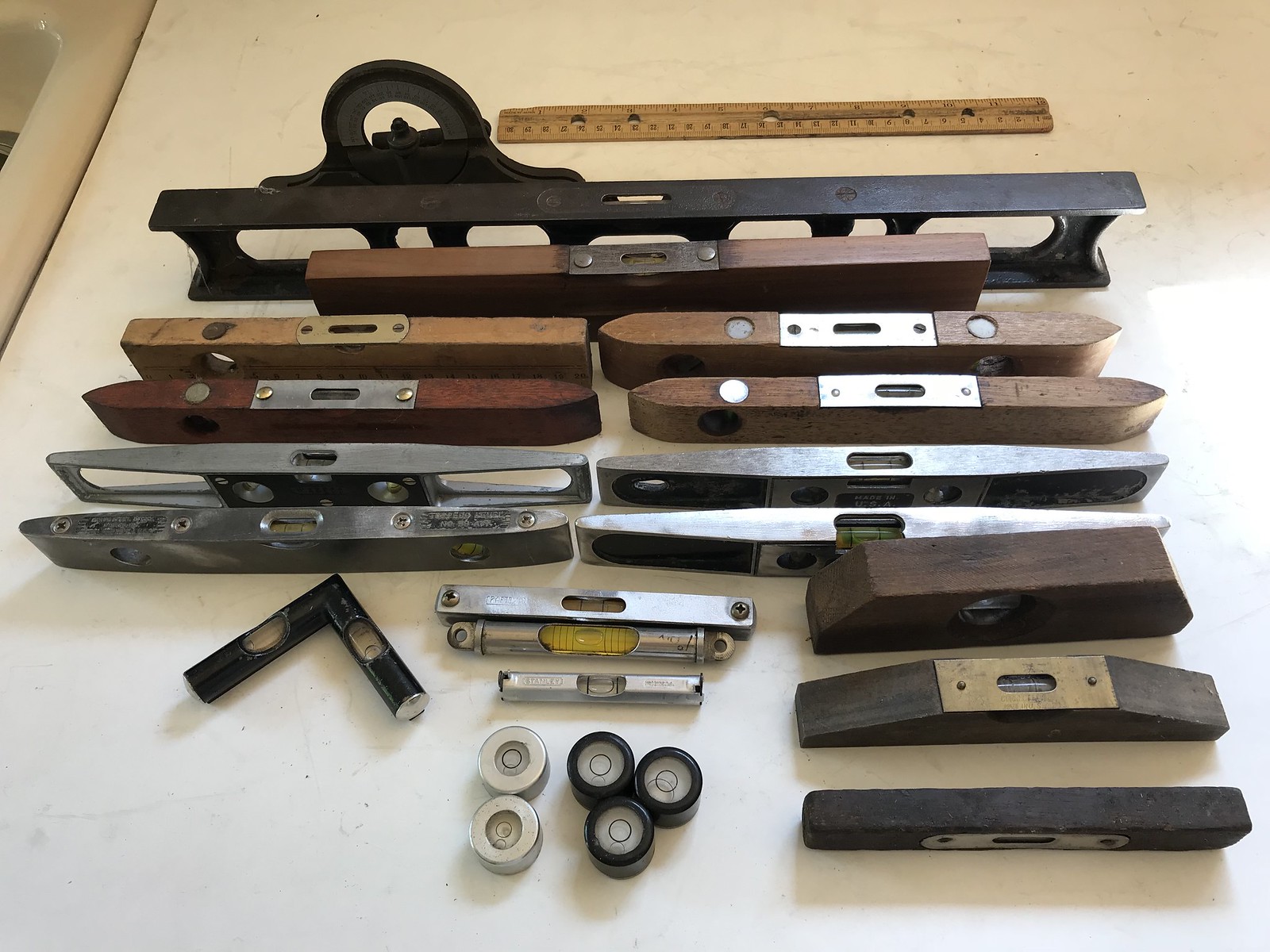This photograph provides an overhead view of a collection of various leveling instruments arranged neatly on a white granite table with a thick tan wooden border. At the very back of the table, there's a conventional ruler, appearing to be longer than 12 inches, followed by an older iron level. The levels, ranging in materials from wood to metal, showcase diverse designs and purposes. The wooden levels exhibit shades from reddish brown to tobacco brown to blonde and feature silver hardware, giving them an antique appearance. Among these tools, notable distinctions include a black, elbow-shaped corner level and a triangular-shaped level missing its base. Additionally, round leveling instruments are scattered in the foreground, comprising three small black circles and two larger white circles, possibly made of plastic or metal. The arrangement consists of longer levels at the back, progressing to shorter ones, and culminating in a variety of shapes and materials, providing a rich historical collection of leveling tools.